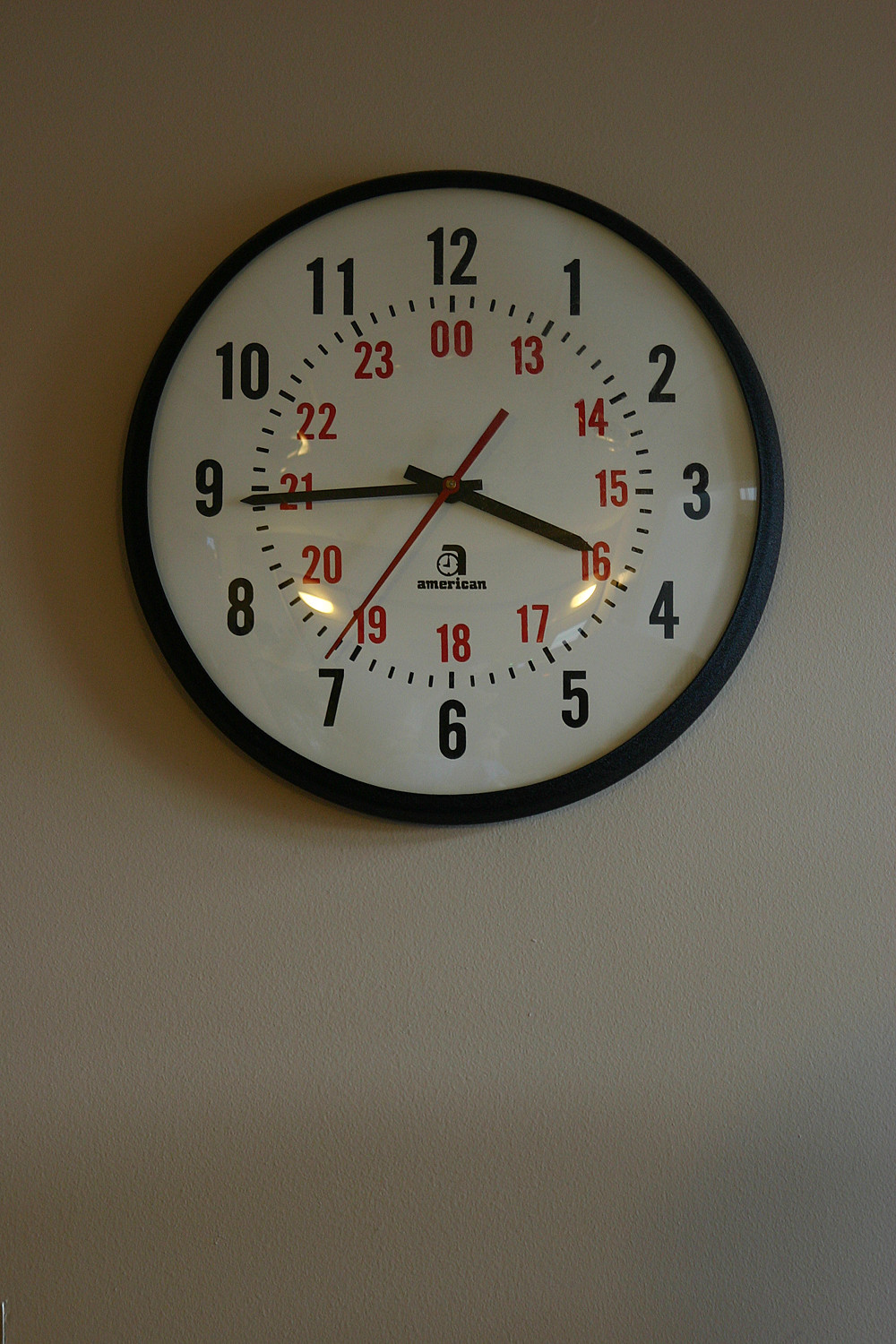The image features a round, simple wall clock mounted on a taupe-colored wall. The clock itself has a black rim framing a white face. The hours are marked with bold black block numbers from 1 to 12, while beneath each of these are smaller red numbers indicating military time from 00 to 23. Oclock's time is currently 3:44. There are three hands on the clock: the hour and minute hands are black, and the second hand is slender and red. Midway down the face, an emblem of a small clock and the word "American" are printed in black text. The clock face is covered by a clear window, which could be made of glass or plastic.